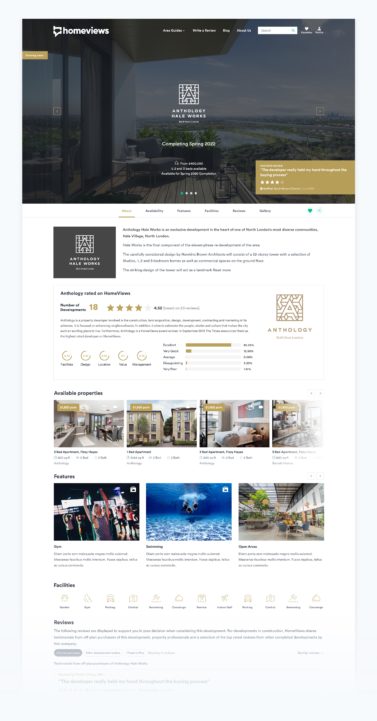In the image, it appears to depict a resort or possibly a high-end apartment complex featuring various luxurious amenities. The overall layout includes several small images, which make it slightly challenging to distinguish specific details, but the impressive facilities suggest it’s a place available for rent. 

In the upper left-hand corner, there’s a section showing "home views," providing a glimpse into the living areas or rooms available at the property. Adjacent to that, a beautiful patio area is prominently displayed, indicating an inviting outdoor space that guests or residents can enjoy.

Notably, in the center of the image, a golden rectangle showcases a rating system. Four out of five white stars are highlighted in gold, signifying a solid 4-star rating. Below this, another review section replicates the rating with four out of five gold-highlighted stars.

Additionally, another segment features review bars, where longer bars likely correlate with better ratings, further emphasizing the high quality of this establishment. 

Other smaller images showcase a variety of scenes, including ocean views and individuals engaged in workouts, further implying a venue rich with amenities. 

Overall, the image represents a resort or luxury apartment complex that offers a comprehensive suite of services and facilities, supported by a commendable rating from its reviews.